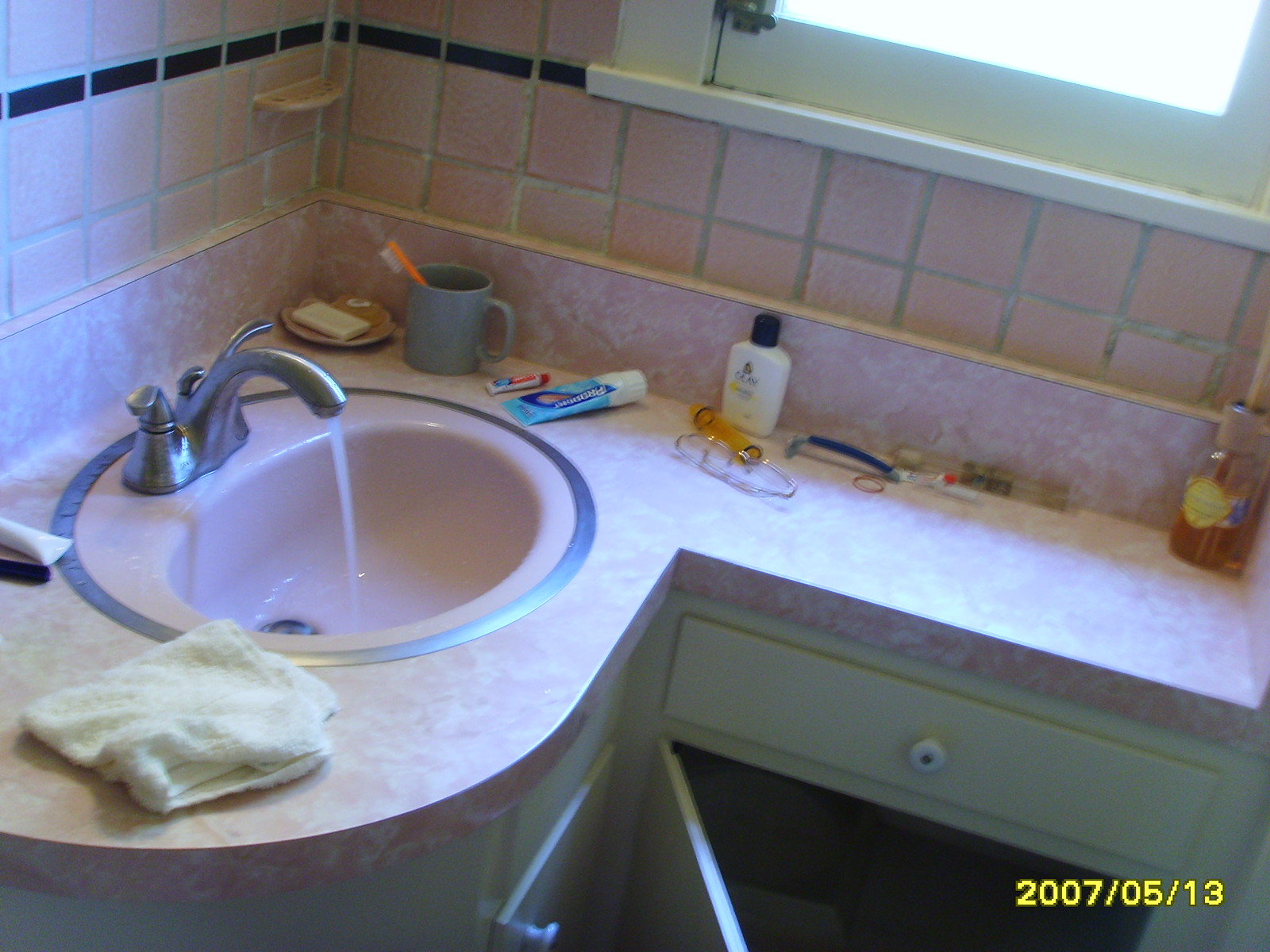In this image of a cozy home bathroom, the focus is on a corner space that showcases a blend of vintage charm and practical details. A window trimmed in white is positioned at the top right, allowing daylight to stream in and illuminate the space. The walls are adorned with pink tiles, interspersed with a single, thin black line that adds a subtle decorative touch. 

The countertop, a marbled pink expanse, complements the hue of the surrounding tiles. At its center lies a pink sink, highlighted by a chrome ring around its edges and a matching chrome faucet, from which water flows steadily. The sink's left side is gently rounded, seamlessly integrating into the corner.

Below the sink, the vanity offers a combination of storage options—a small drawer and a cabinet with its door ajar. 

The countertop hosts an array of personal care items: a bottle of Olay face lotion, a tube of toothpaste, a small miscellaneous tube, a razor, possibly a bottle of cologne, a soap dish containing soap, a cup holding a toothbrush, another tube to the sink's left, and a washcloth, each contributing to the lived-in feel of the space.